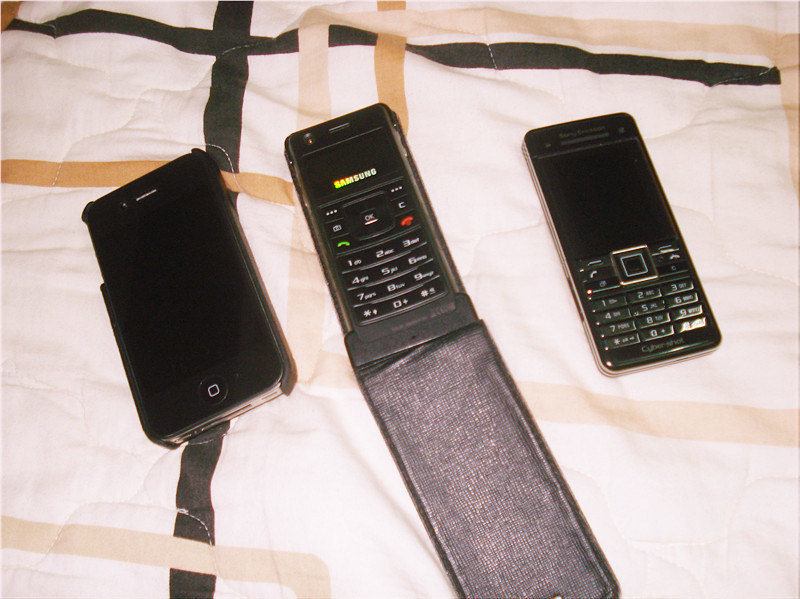The image features three early-model cell phones laid out on what appears to be a comforter with distinctive black, amber, beige, and cream stripes. The comforter has visible stitching and gives a textured canvas for the phones, contributing to a nostalgic setting. On the left is an early model iPhone, identifiable by its home button and older wide charging port, typical of iPhones from the late 2000s. In the middle is a Samsung phone, noted for its minimal screen size, characteristic of early flip phones. On the right is another older phone with a larger screen and physical keyboard, suggesting it might be a transitional model from the early 2000s. The iPhone and the third phone are turned off, while the Samsung is powered on. All three phones are placed in an upright position, emphasizing their varied yet outdated designs.